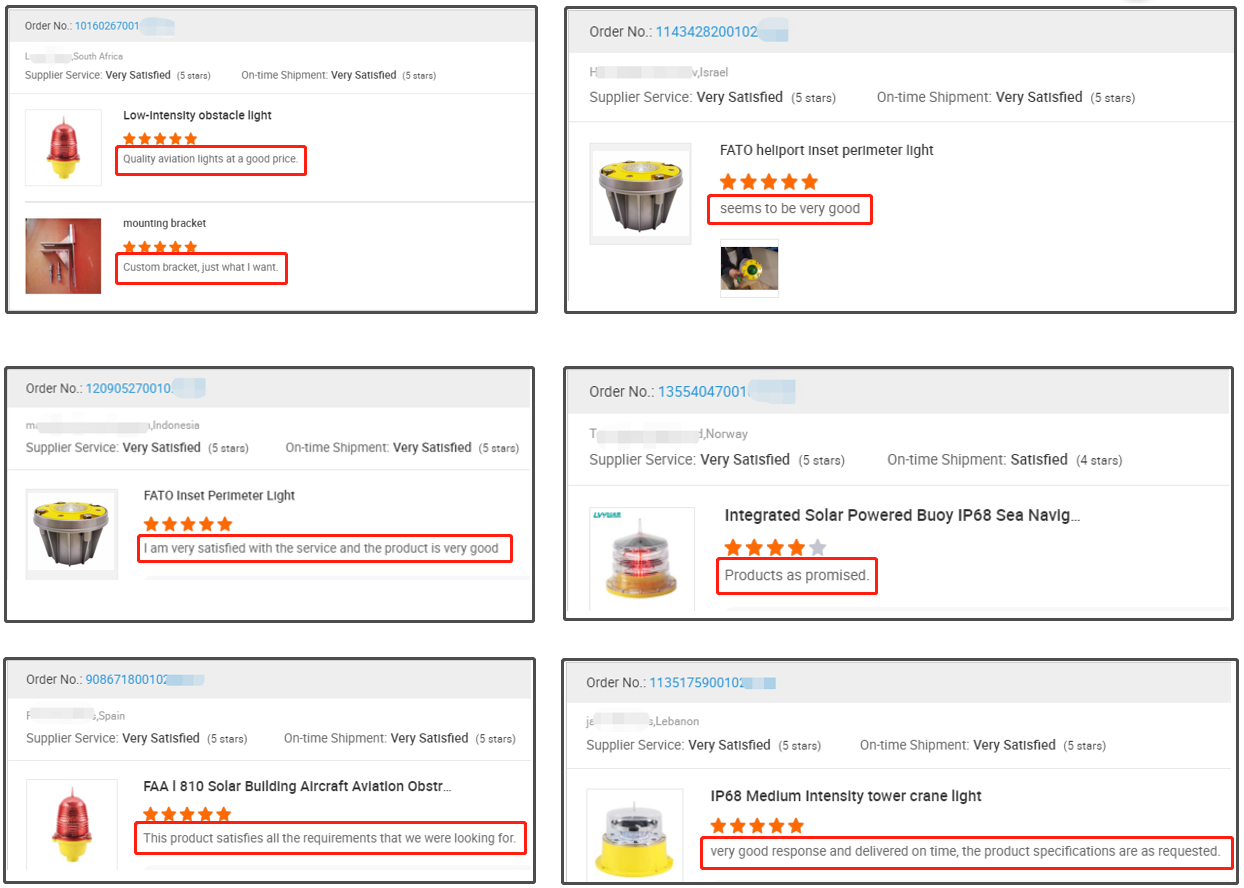This screenshot captures six distinct orders, each outlined in black and presented within rectangular boxes. The rectangles are arranged in two columns: the left column features three identical-size rectangles stacked vertically, while the right column has three wider rectangles, with the bottom one being slightly wider than the other two.

1. **Upper Left Order: Low Intensity Obstacle Lighting**
   - Rating: ⭐⭐⭐⭐⭐
   - Description: Appears to be an emergency hazard light, some areas outlined in red.
   - Comments:
     - "Quality aviation lights at a good price, with a five-star rated mounting bracket."
     - "Custom bracket, just what I wanted."

2. **Middle Left Order: FATO Insert Perimeter Light**
   - Rating: ⭐⭐⭐⭐⭐
   - Comments:
     - "Supplier service is very satisfactory."
     - "Very satisfied with the service, the product is very good."

3. **Bottom Left Order: Aviation Outdoor Light**
   - Rating: ⭐⭐⭐⭐⭐
   - Comments:
     - "This product satisfies all the requirements we were looking for."

4. **Upper Right Order: FATO Heliport Insert Perimeter Light**
   - Rating: ⭐⭐⭐⭐⭐
   - Comments:
     - "Seems to be very good."

5. **Middle Right Order: Integrated Solar-Powered Buoy, IP68C Navigation**
   - Rating: ⭐⭐⭐⭐
   - Comments:
     - "Product delivers as promised."

6. **Bottom Right Order: IP68 Medium Intensity Tower Crane Light**
   - Rating: ⭐⭐⭐⭐⭐
   - Comments:
     - "Very good response and delivered on time. The product specifications are as tested."

Each rectangle includes a thumbnail image of the respective light or bracket, offering a visual reference for the described items.